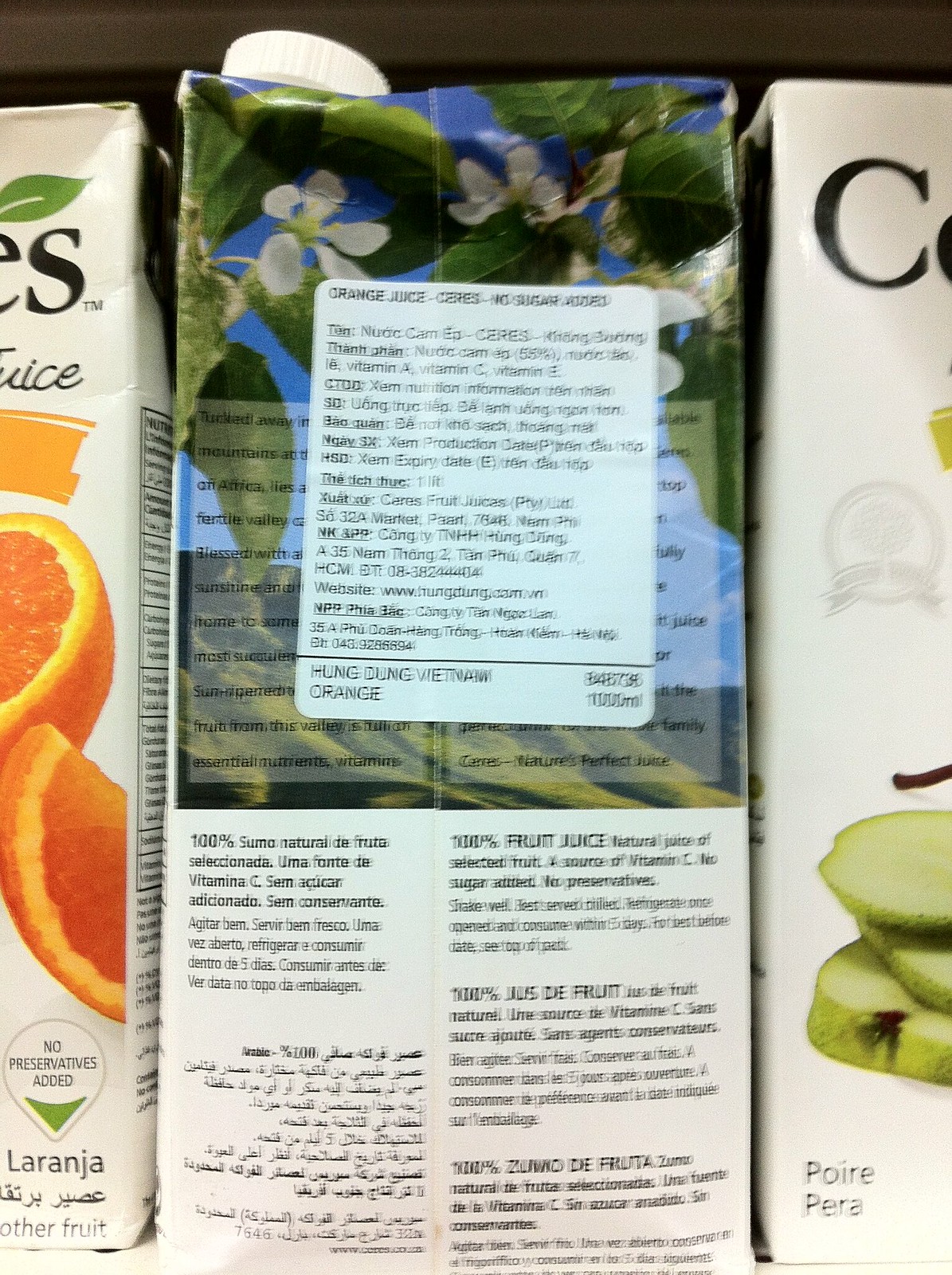The image displays three boxes of beverages, possibly flavored waters or juices. The box on the left prominently features oranges and the word "juice" on its label. The box on the right appears to contain either pear or apple juice, with the label showcasing a pear and starting with the letter "C." The bottom text on this box is unclear, but includes the fragment "pera." The box in the middle is turned backward, making the label difficult to fully discern. However, it includes the phrase "100% fruit juice" and seems to contain writing in another language, possibly Arabic.